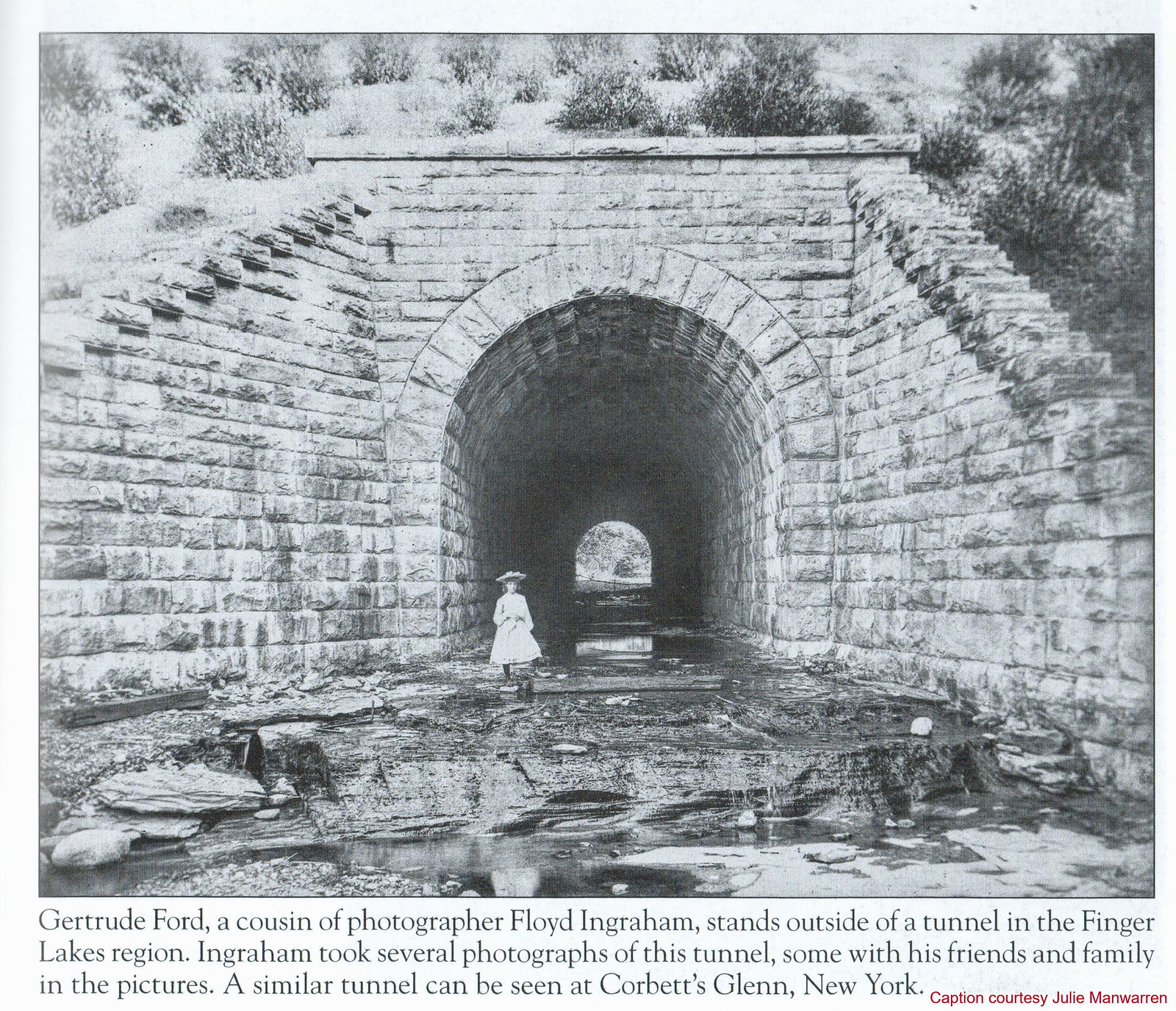This vintage black and white photograph captures the entrance of a large stone tunnel, possibly used for trains, located in the Finger Lakes region. At the forefront stands Gertrude Ford, a cousin of photographer Floyd Ingraham. She is dressed elegantly in a white or light-colored dress, stockings, and a hat, indicative of the late 19th to early 20th century style. The ground in front of the tunnel appears muddy, and there are bushes behind the structure. The caption at the bottom of the photograph, written in a serif font, reads: "Gertrude Ford, a cousin of photographer Floyd Ingraham, stands outside of a tunnel in the Finger Lakes region. Ingraham took several photographs of this tunnel, some with his friends and family in the pictures. A similar tunnel can be seen at Corbett's Glen, New York." The words "caption courtesy of Julie Mann Warren" are printed in red, in a sans-serif font reminiscent of Arial.